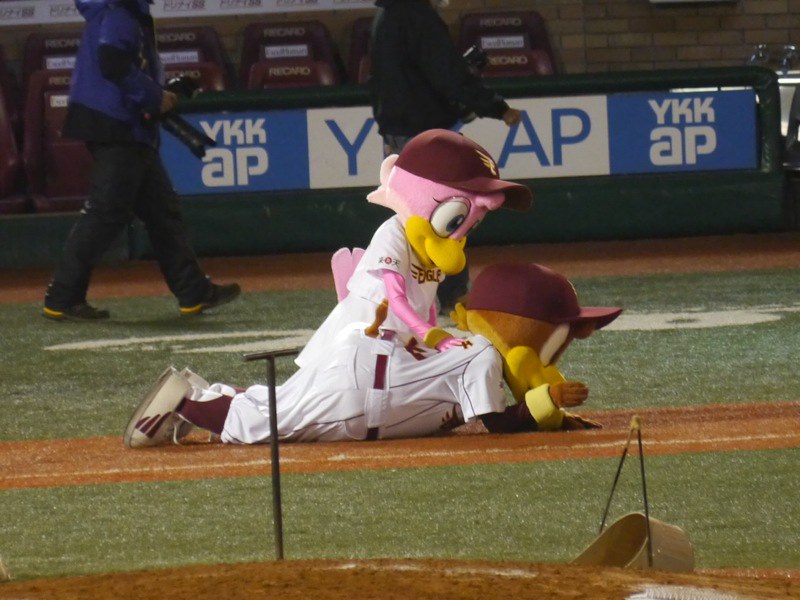The image captures a lively scene at a baseball game in an outdoor stadium during the day. At the center of the image are two colorful mascots seemingly engaged in playful antics. One, a pink female bird wearing a baseball jersey with the word "Eagle" on it, is standing over the other, a brown male bird who is lying on the ground. Both mascots are dressed in baseball uniforms complete with caps, and their yellow beaks are prominently visible.

Surrounding the central action, the setting features a large, flat, grassy field with a few dirt mounds scattered across it, hinting at its use as a baseball field. In the background, there are several spectators seated and a couple of photographers walking past, though their heads are cut off at the top of the image. The photographers are distinguishable by their attire, one in black pants and a blue jacket, and the other in a black jacket. 

A sign bearing the logo "YKKAP," a likely indication of the Japanese firm sponsoring the event, is prominently displayed near the seats in the background. The overall color scheme includes a variety of hues such as green for the grass, brown and pink for the mascots, and additional colors from the spectators and photographers.